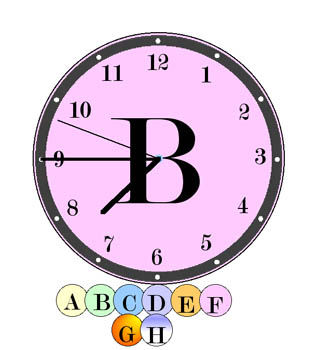The image depicts an artistic, computer-generated clock with a round face that has a pinkish-purple (lavender/mauve) tint. At the center of the clock is a large black letter "B", from which the hour, minute, and second hands emanate. The clock displays the time as approximately 7:45:49. Surrounding the numbers on the clock face is a decorative gray circle accented with white dots at each number intersection. Beneath the clock, there is an array of colorful bubbles containing the letters A through H, each in a different color: A in yellow, B in green, C in blue, D in purple, E in orange, F matching the mauve color of the clock face, G in dark orange, and H in another shade of purple.